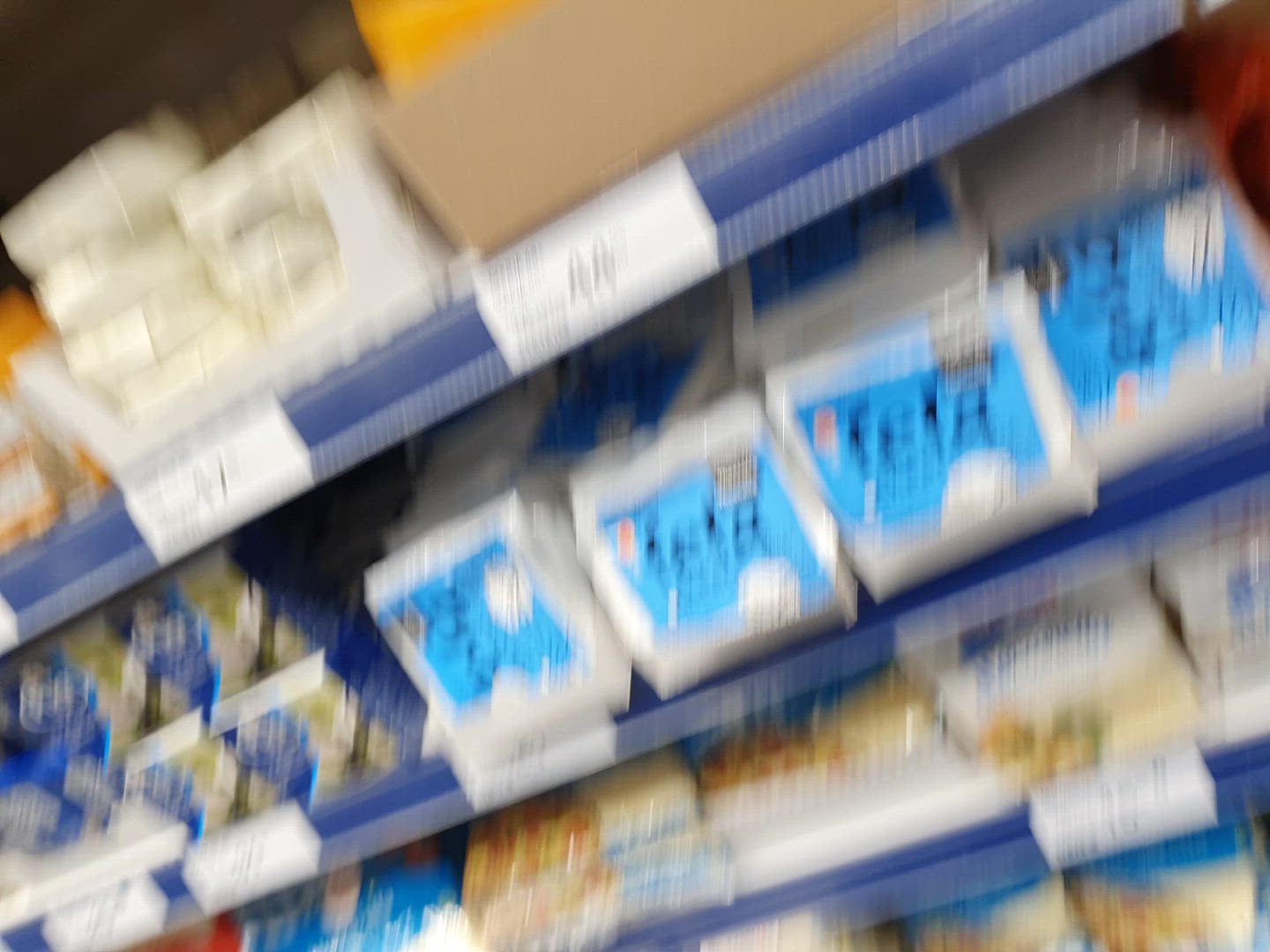A blurry, slanted photograph of grocery store shelves reveals a disorganized scene, slightly tilted from the lower left to the upper right. The blue-colored shelves, arranged in three rows, display various indistinct items, each marked with price stickers. On the middle shelf, four noticeable squares feature Feta cheese labels—primarily white with prominent blue and darker blue text reading "Feta." Other product labels are generally indiscernible due to the blurriness, though some appear white, while a few stand out in blue and yellow hues, with more orangey-brown labels located on the bottom shelf. A cardboard box is seen resting on one of the top shelves, positioned towards the right side.